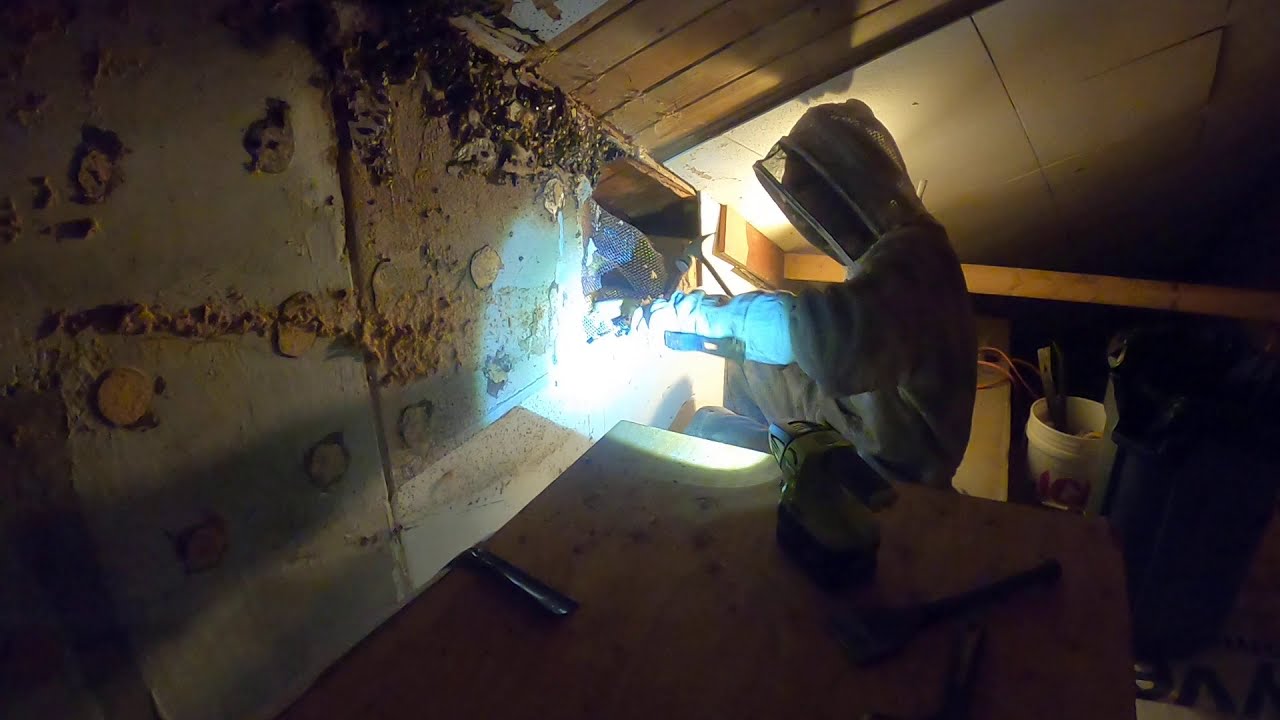The image depicts a man dressed in full protective gear, including a white beekeeper's outfit, blue gloves, and a netted mask over his face. He appears to be in an attic-like area or shed with a slanted ceiling, surrounded by various tools, including a hammer in his right hand and an industrial-sized flashlight illuminating his workspace. The environment is rough, with visible wooden beams and exposed brown wood paneling amidst white ceiling panels. He seems to be working on or repairing the structure, possibly dealing with a beehive or some other issue, as there are signs of bees and nests on the wall. Patches on the wall and traces of glue suggest he has removed some paneling. Additionally, a bucket labeled with the letters "AC" and filled with tools is visible in the background, alongside a drill lying on a table or the floor to his left. The scene is dimly lit, except for the direct light from his headlamp, making it difficult to determine the exact nature of his task, though it clearly involves detailed and cautious work.